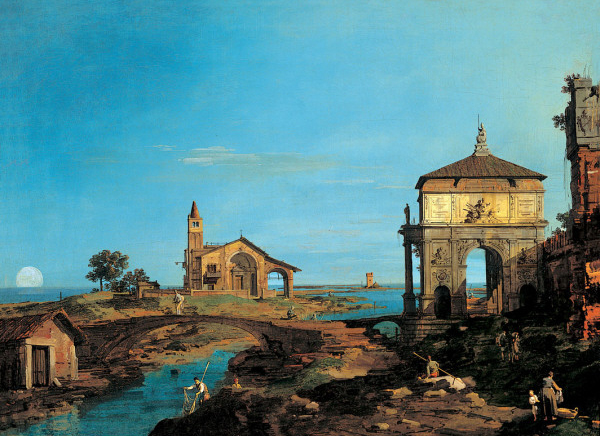In this highly detailed and realistic painting, reminiscent of a photograph, the scene captures a tranquil village set along a serene waterway. Dominated by an expansive, light blue sky peppered with delicate white clouds, the moon is subtly setting on the left side, casting a soft glow over the scene. At the bottom left corner, a man with a fishing net and pole focused on his catch adds a touch of daily life to the image. The waterway, possibly part of a canal or stream, is spanned by a quaint, small bridge approximately 10 to 15 feet tall, with a solitary figure standing upon it, adding depth to the composition.

To the right side of the foreground, a woman and a child, possibly engaged in folding laundry, lend a homely touch to the scene. Nearby, another fisherman can be seen while two more figures appear to traverse towards a large arched structure, further enhancing the narrative of village life.

The background is enriched with two prominent old-style buildings, one centrally located and the other towards the right side, both meticulously detailed and seemingly historic. Complementing these is a building with a tower, nestled among a few trees, creating a picturesque backdrop. This evocative painting masterfully captures a bygone era, transporting viewers to a peaceful village by the water, woven together with the simplicity and charm of everyday life.